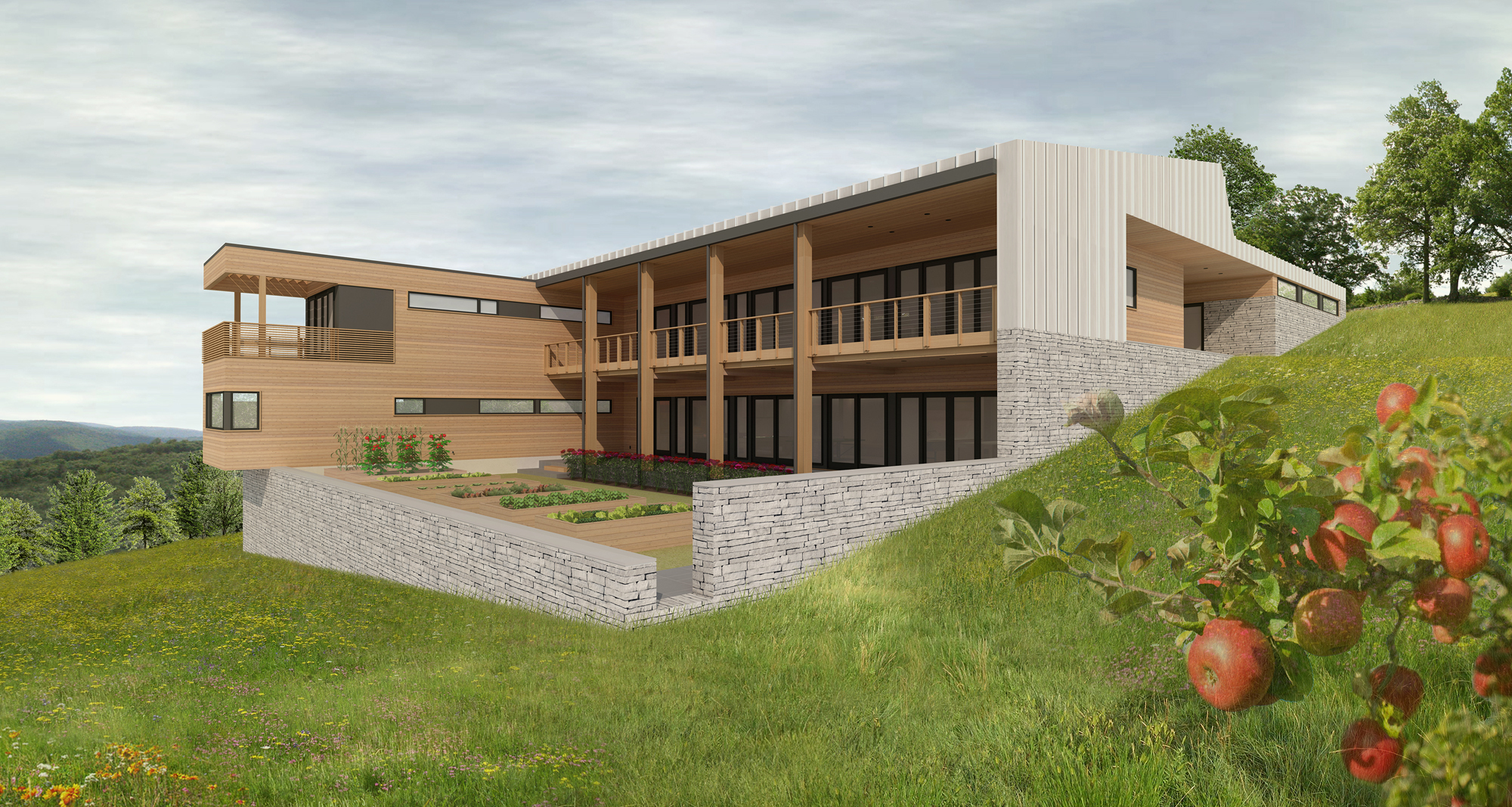This is an outdoor image of a computer-generated, modern house, intricately built into a hillside. The house features a distinct combination of wood and stone, with its two floors nestled seamlessly into the green landscape. On the left side, the house is characterized by a brown wooden exterior and stone walls. The lower level boasts large windows, while the upper level includes a balcony with a minimalist railing.

Emerging from the slope of the hill, the structure blends naturally into its surroundings. The foreground showcases lush green grass, while to the right, a tree with branches laden with red apples adds a touch of natural charm. Further up the hill, there is an area covered with more trees, creating a scenic backdrop. The backyard also includes a well-kept garden area with three distinct patches of greenery.

In the background, a series of rolling mountains under a blue sky dotted with patches of clouds frame the scene, enhancing the serene and picturesque setting. The image perfectly captures the harmonious blend of modern architecture and the tranquil beauty of nature.